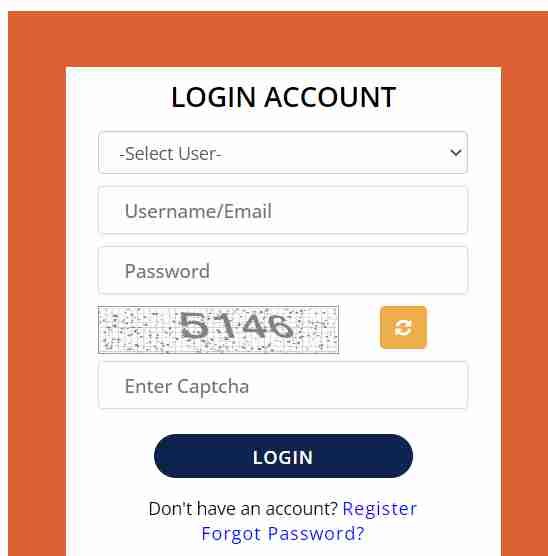The image depicts a login screen with a muted, orangey-peach rust-colored background. Central to the screen is a prominent white rectangle framing the login interface. At the top of this rectangle, bold black text reads "Login Account." 

Below this heading is a dropdown menu labeled "Select User," followed by fields designated for "Username/Email" and "Password." Beneath the password field lies a CAPTCHA—a series of numbers, specifically "5146," set against a grungy, textured background. Adjacent to the CAPTCHA is a small orange button adorned with two rotating circular arrows, which users can click to refresh the CAPTCHA if it's unreadable.

Following the CAPTCHA section is an input field where users can type the provided numbers. At the bottom of the interface, a large, blue, capsule-shaped button labeled "Login" prominently invites users to proceed.

Supplementary options include a hyperlink in blue text for users who "Forget Password?" and another for those who "Don't have an account? Register," directing them to registration via clickable blue text.

The overall image quality appears heavily compressed, with noticeable grungy artifacts typical of a low-quality JPEG file, despite the simplicity and limited color palette of the design elements.